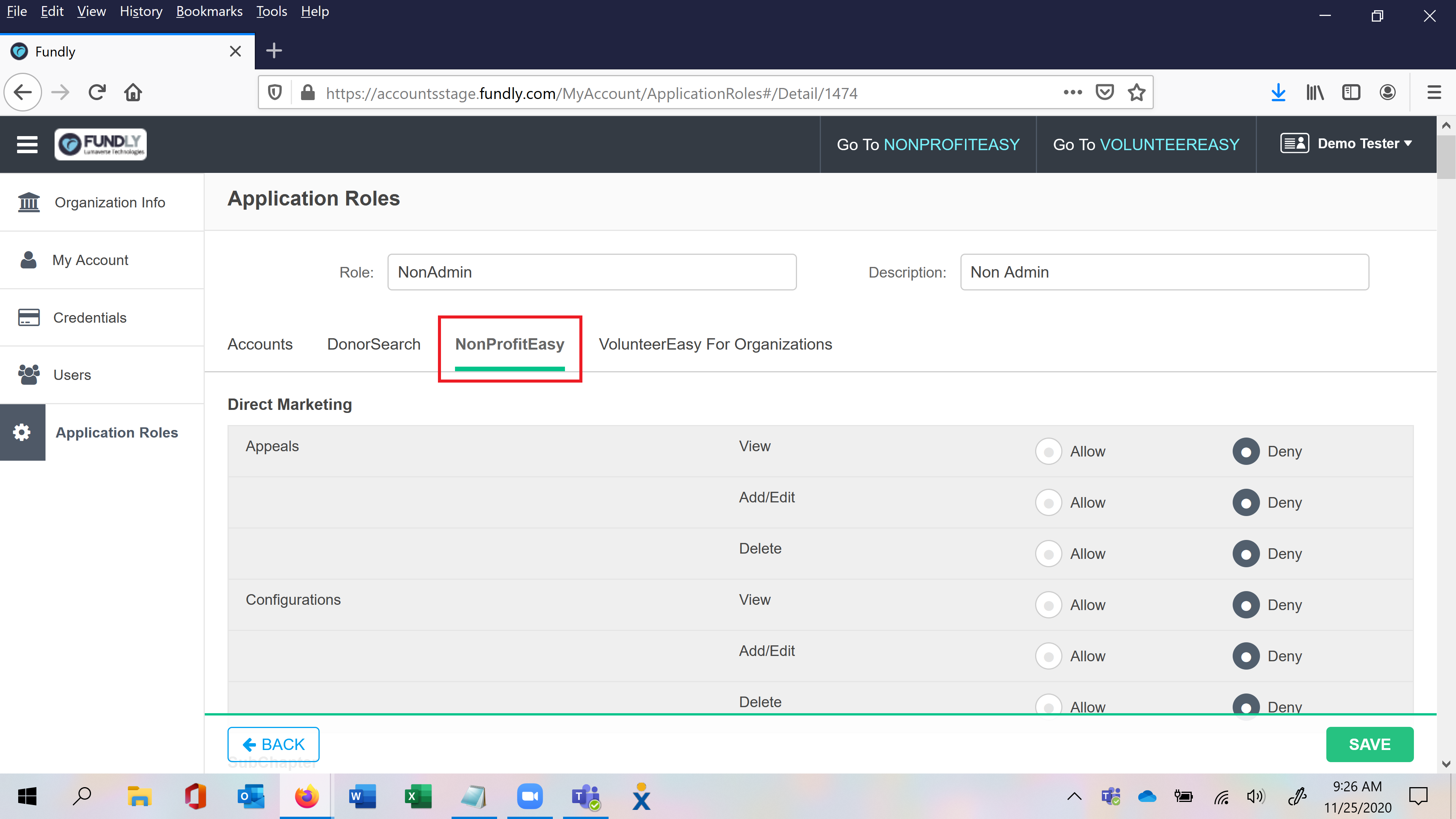This image is a screenshot of a Firefox browser window open on a Windows computer. The browser's menu bar at the top includes options for File, Edit, View, History, Bookmarks, Tools, and Help. The webpage displayed is from a website called Fundly. At the top of the Fundly site, there's a navigation menu with options to access 'Non-Profit Easy,' 'Volunteer Easy,' and a 'Demo Tester.'

On the left side of the Fundly page, a vertical menu lists clickable sections such as 'Organization Info,' 'My Account,' 'Credentials,' 'Users,' and 'Application Roles,' with 'Application Roles' currently selected. The active section details the following:
- Role: Non-admin
- Description: Non-admin

The active role includes access permissions for various features like 'Accounts,' 'Donors,' 'Search,' 'Non-Profit Easy,' and 'Volunteer Easy for Organizers.' The 'Non-Profit Easy' feature is highlighted with a red rectangular box and underlined in green, marked as 'Direct Marketing.'

Below it, there is a gray box with sub-sections labeled 'Appeals' and 'Configurations.' Both of these options have settings for 'View,' 'Add,' 'Edit,' and 'Delete,' each accompanied by radio buttons for 'Allow' or 'Deny.' In the screenshot, all permissions are set to 'Deny,' indicated by filled-in circles next to the 'Deny' options.